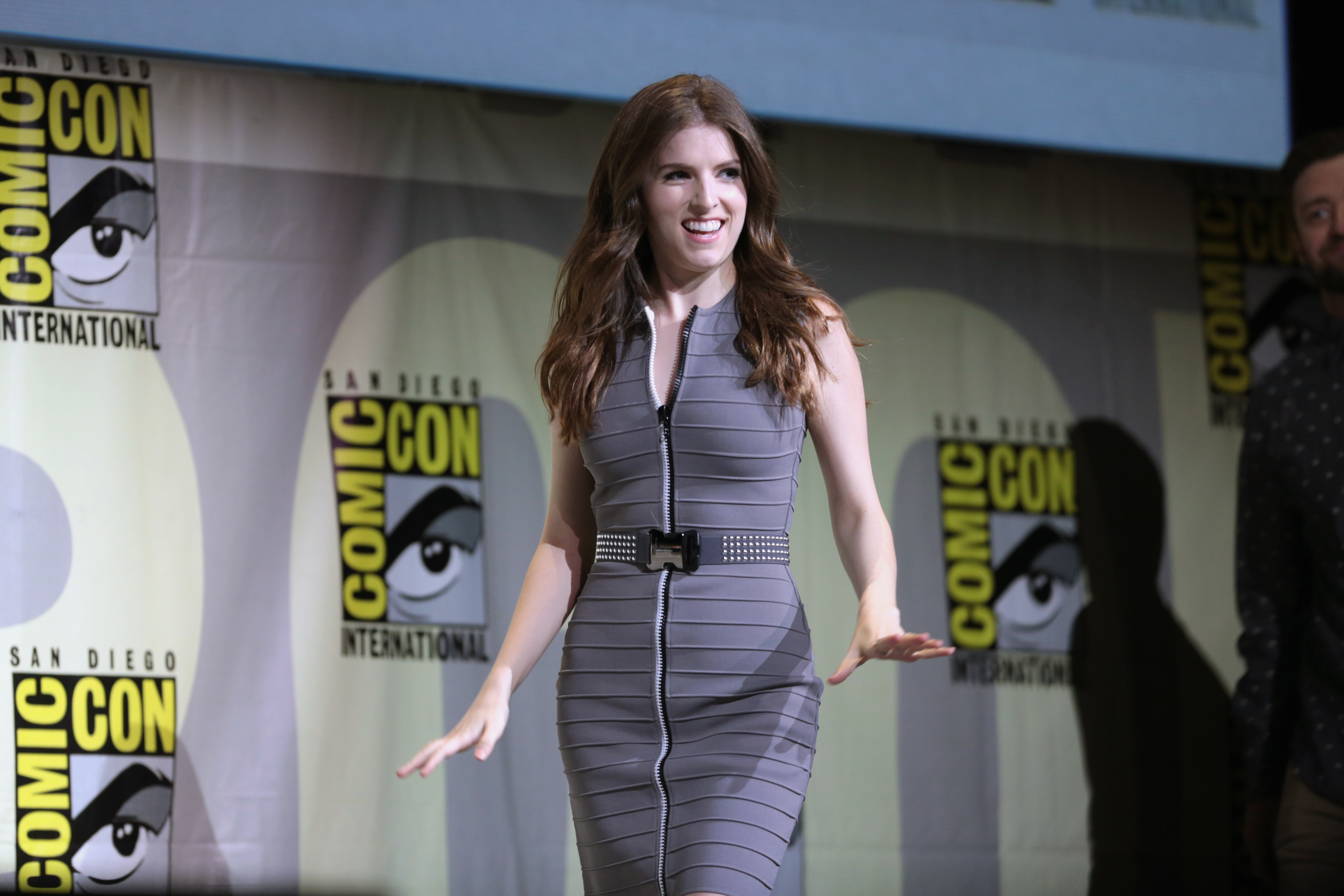In this vibrant photograph taken at Comic-Con International, a familiar yet unnamed actress stands confidently at the center of the stage. She is wearing a form-fitting, sleeveless gray dress with thin, raised ridges made from the same material, giving it a textured appearance. A black zipper runs down the front of the dress, unzipped to mid-chest level. The outfit is accessorized with a gray belt adorned with silver studs and a black buckle around her waist. She appears to be engaging with the audience or responding to someone, her dark hair cascading just below her shoulders, as she looks animatedly towards the right side of the photograph. Both her arms are extended to her sides, with her hands spread out flat, palms facing downwards. The backdrop is a curtain wall adorned with a logo that repeats five times, featuring yellow text that reads "Comic-Con" vertically and "International" in black text, all set against a background of gray, yellow, and light gray hues. Additionally, there is a partially visible man in the background to the right, wearing a black and white dotted shirt, adding context to the bustling atmosphere of the event.